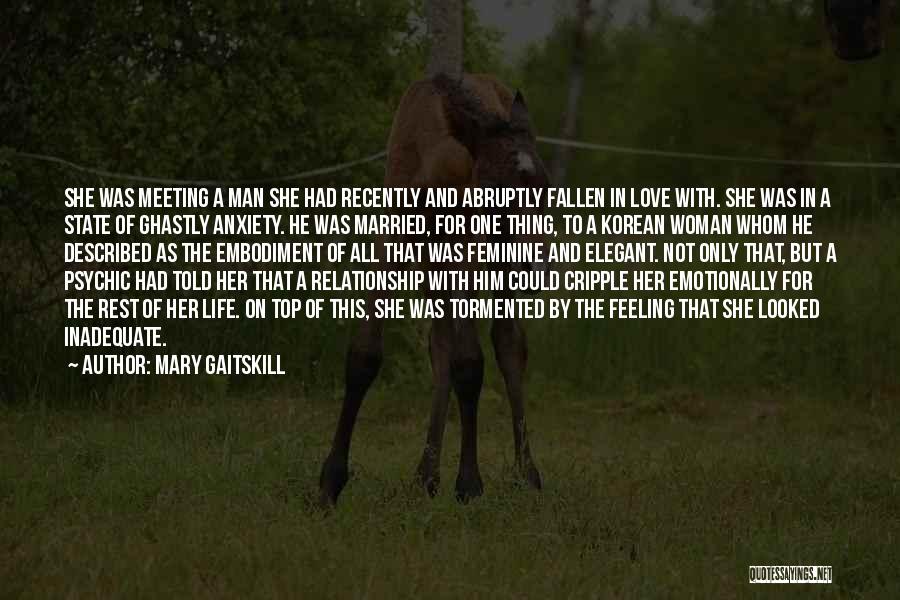The image features a faint, blurred photograph of a brown horse with a white spot on its head, standing in a field enclosed by a fence, with trees and grass visible in the background. The entire picture has a darkened overlay with a significant portion of the image occupied by a block of white, all-caps text. The text reads: "SHE WAS MEETING A MAN SHE HAD RECENTLY AND ABRUPTLY FALLEN IN LOVE WITH. SHE WAS IN A STATE OF GHASTLY ANXIETY. HE WAS MARRIED, FOR ONE THING, TO A KOREAN WOMAN WHOM HE DESCRIBED AS THE EMBODIMENT OF ALL THAT WAS FEMININE AND ELEGANT. NOT ONLY THAT, BUT A PSYCHIC HAD TOLD HER THAT A RELATIONSHIP WITH HIM COULD CRIPPLE HER EMOTIONALLY FOR THE REST OF HER LIFE. ON TOP OF THIS, SHE WAS TORMENTED BY THE FEELING THAT SHE LOOKED INADEQUATE." At the bottom of the text, credit is given to author Mary Gaitskill, and in the bottom right-hand corner appears the watermark "quotesayings.net."